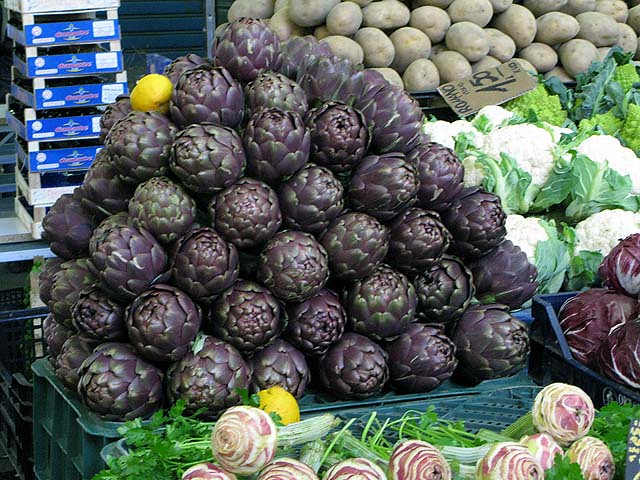The photograph captures a bustling market, teeming with an array of fresh produce meticulously arranged in crates. Dominating the foreground is a vibrant collection of vegetables, highlighted by an intriguing purple and green layered vegetable that some might mistake for an exotic variety like dragon fruit or a distant cousin of an eggplant, though its exact identity remains elusive. Surrounding this centerpiece, there are piles of cauliflower heads and root vegetables, possibly green onions or radishes, adding to the earthy palette. In the background, heaps of potatoes fill up several crates, providing a rustic contrast to the more colorful produce. Various crate colors, ranging from greenish-blue to black, create a patchwork effect on the marketplace floor. A slightly askew cardboard sign, situated near the cauliflower and potatoes, features partially legible text reading "RO something 150," hinting at prices for the goods on display. The scene, framed within a side street market, exudes an authentic, fresh-from-the-farm atmosphere, inviting onlookers to explore the bounty of produce available.